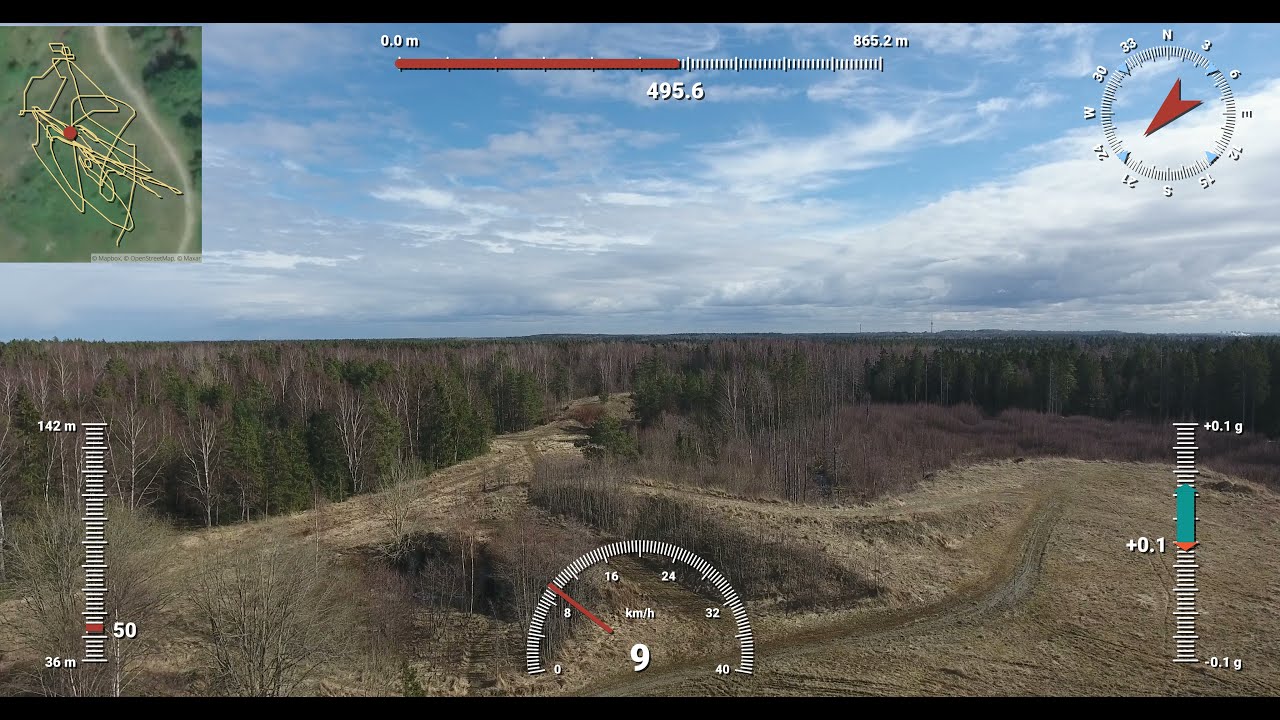The image shows what appears to be a drone's perspective, captured mid-flight over a sparse forest landscape characterized by bare tree trunks, the occasional green pine, and patches of yellowish grass, indicating the fall season. The sky occupies the upper half of the frame, a light blue canvas with scattered cirrus clouds. On the bottom half, a variety of on-screen overlays and navigation data are visible. Central to the bottom is a speedometer indicating the drone is flying at 9 kilometers per hour, featuring a red dial pointing to the left and a scale ranging from 0 to 40 KMH. Flanking the speedometer, there are altitude gauges: the left one includes a small red rectangle with a reading of 36M at the bottom and 142M at the top, while the right one shows a vertical bar with white stripes, labeled with a turquoise blue rectangle near the top, and markings of 0.1G at the top and -0.1G at the bottom. An inset map in the top left corner displays a series of yellow-gold squiggly lines with a red dot in the center, presumably illustrating the drone's flight path. The upper middle section provides the altitude reading of 495.6 meters. On the top right, there's a compass indicating a southwest direction. The overall scene resembles a sophisticated navigation interface superimposed onto a desolate, forested backdrop.